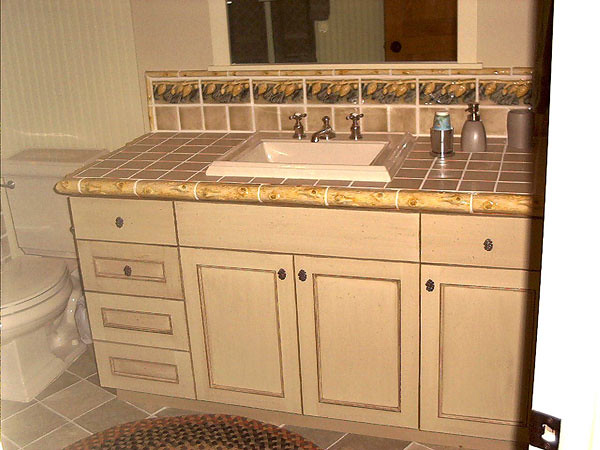The image depicts a bathroom with a variety of detailed features. Starting from the bottom, the floor is laid with square tiles in two different shades of gray. A small portion of a braided rug, featuring green and rust colors, is visible. To the far left of the image is a modern white toilet. Directly adjacent to the toilet, with only a few inches of space in between, is a large vanity sink. 

The vanity includes three cabinets and four drawers on the left side, with an additional drawer above one of the cabinets on the right side. The countertop is tucked under smooth, rounded tiles that are copper-colored. The sink itself is white and modern in design, featuring a single spout and two faucet handles in a bronze finish. 

On the vanity, there is a dispenser for disposable cups and another dispenser, likely for lotion. Above the sink, the backsplash consists of brownish tiles with a decorative tile strip above it. A mirror with a white border hangs above the backsplash, completing the elegant and functional design of this bathroom.